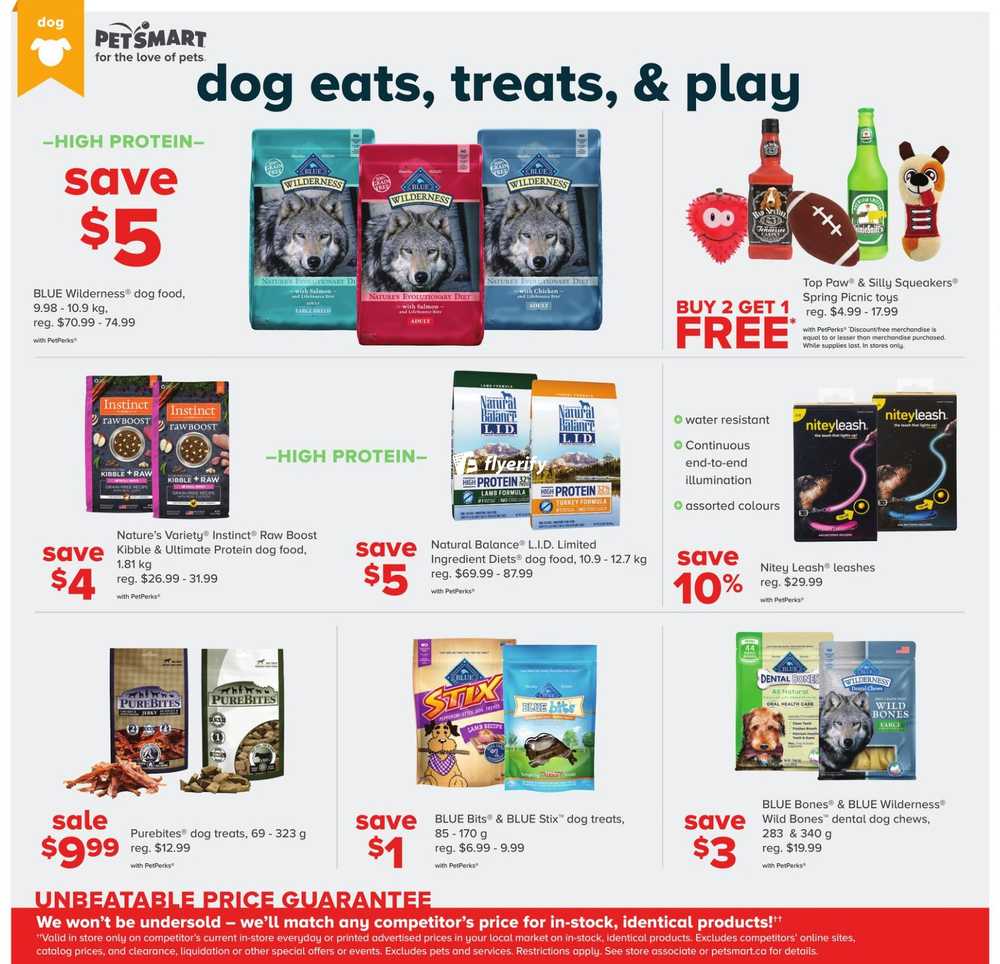The image showcases a sales flyer with a gray background. At the top left corner, there is an orange ribbon with pointed edges at the bottom that features the word "DONG" and a silhouette of a dog's head. To the right of this, the PetSmart logo appears, accompanied by the slogan "For the Love of Pets." Below the logo, the phrases "Dog Eats, Treats, and Plays" are prominently displayed.

The flyer highlights three bags of dog food situated beneath the tagline. The bag on the left is bluish-gray, the one in the middle is burgundy, and the one on the right is a purplish blue. Each bag features an image of a husky on the front. To the left of these bags, the text "High Protein, Save $5, Blue Wilderness Dog Food" is displayed.

Further down, the flyer displays two additional bags of dog food on the left side. These bags are black with a purple border and an orange logo at the top. Adjacent to these bags, the text "High Protein" is visible, followed by "Nature's Variety, Instinct, Raw Boost Mixers, and Ultimate Protein Dog Food," along with a note that says "Save $4."